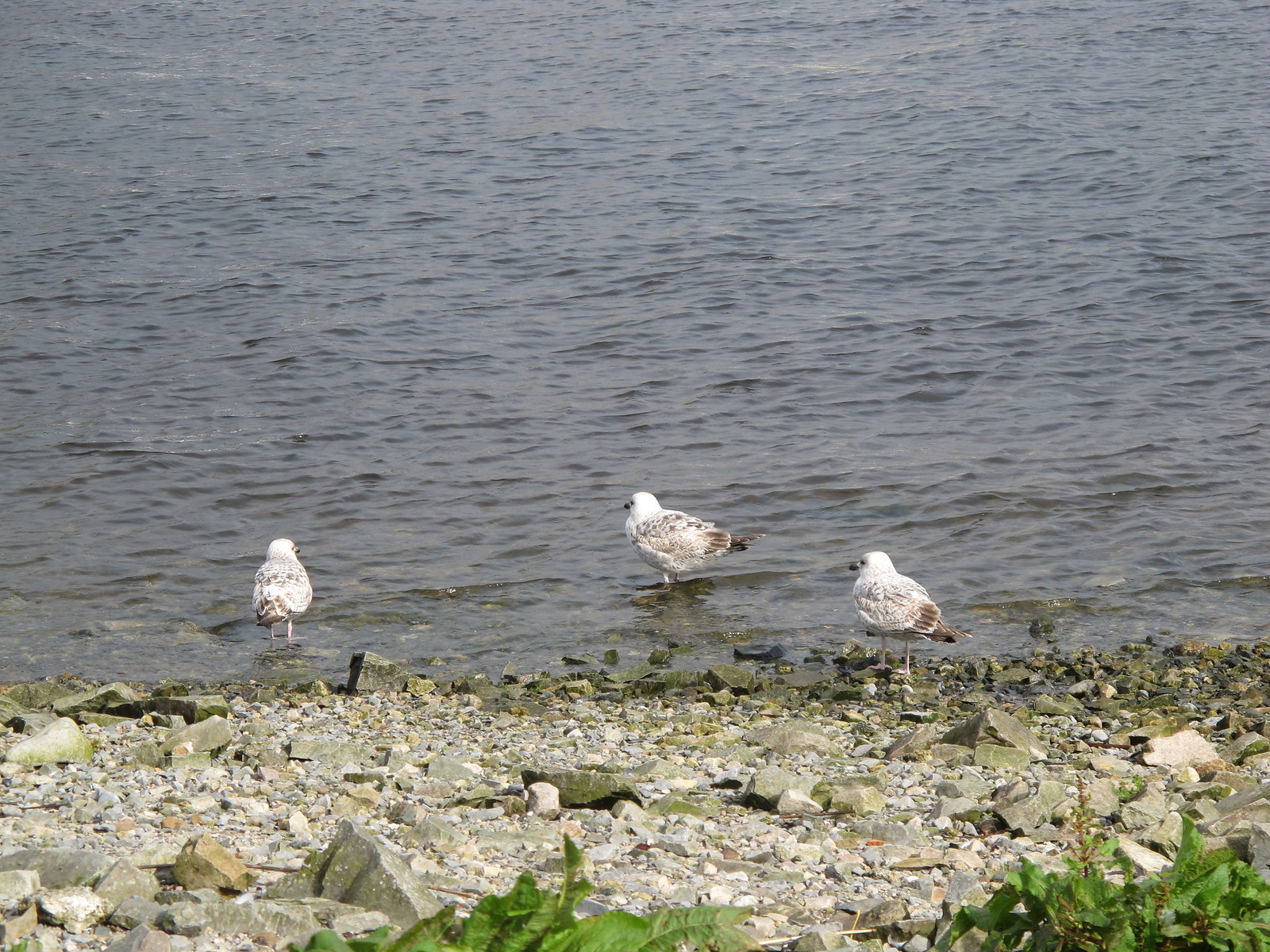This photograph captures a quiet, overcast day at the edge of a pond. The shallow, murky water appears almost still, with only slight ripples disturbing its grayish-brown surface. Along the rocky shoreline, variously sized rocks and some patches of vegetation are visible. In the foreground, three white birds with dark beaks stand in the shallow water. Their plumage is predominantly white with brown specks, and their wings and tail tips show more prominent brown feathers. The birds' dark eyes are noticeable against their white heads. The overall scene exudes a calm, natural beauty despite the cloudy weather and the pond's murky water, highlighting the simple yet captivating presence of the birds and their environment.